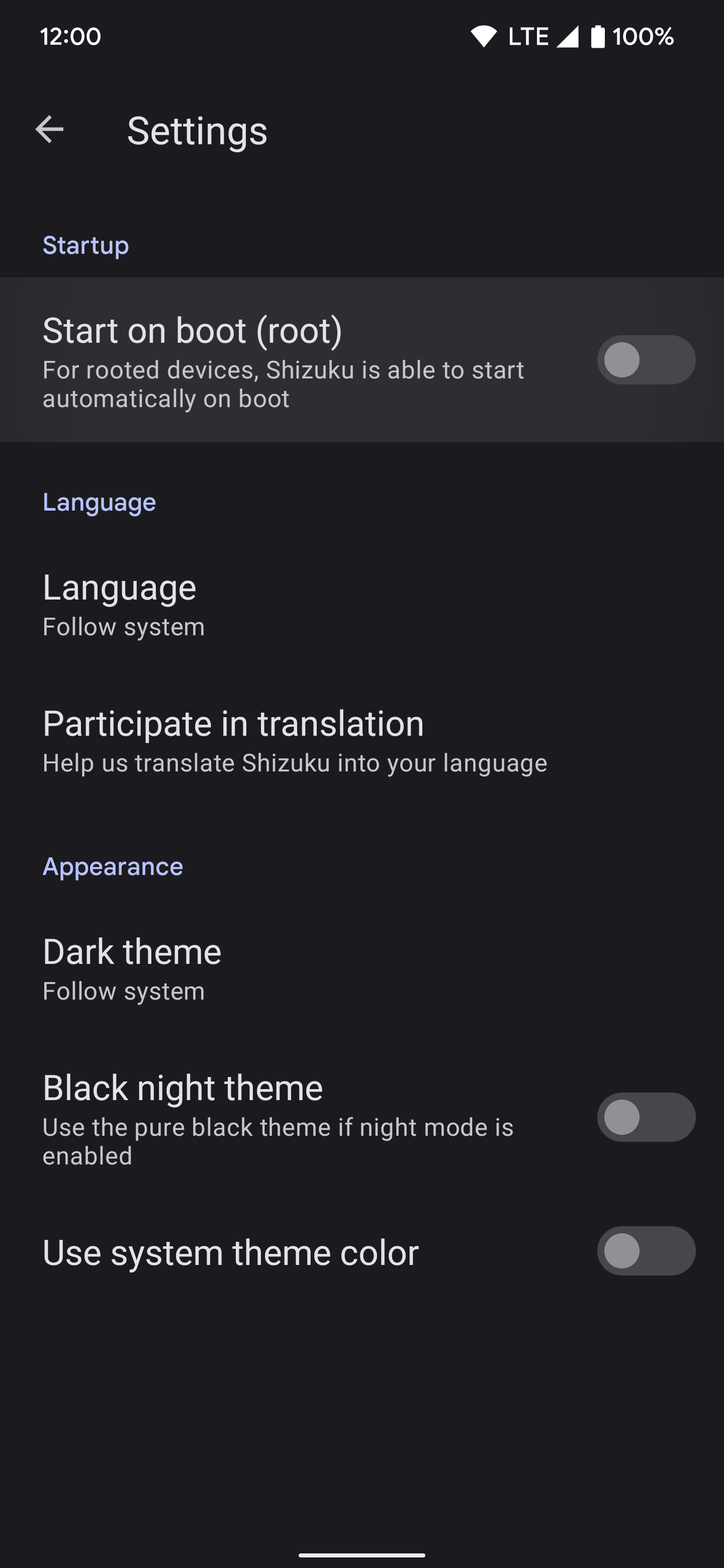**Detailed Caption:**

The image showcases the settings interface of the Shizuku app on a smartphone. The top status bar displays "12 LTE" for network connectivity, the Wi-Fi symbol, a 100% battery indicator, and a gear icon representing the settings menu. 

The main screen provides several configuration options for routed devices. Notably, Shizuku is highlighted for its capability to start automatically on boot. The settings include a "Toggle Language" option, which allows users to choose whether the app's language follows the system language. 

There is a call to action inviting users to "Participate in Translation" to help translate Shizuku into different languages. 

Under the "Appearance" section, users can switch between the dark theme, which follows the system's settings, and a "Black Night Theme," using a pure black background when night mode is enabled. The interface also offers a toggle for "Use System Theme Color." The entire settings page is depicted with a black background and white text, divided by a gray line at the bottom and center of the screen.